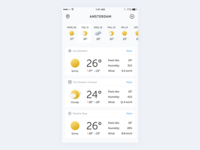A screenshot of a weather app displayed on a cell phone screen, encapsulated within a larger light gray square. At the top of the screenshot, status indicators such as the service bar on the left, the current time in the center, and the battery percentage on the right are visible. The location label of the weather forecast is also present but not fully readable due to blurriness.

The forecast section showcases weather predictions for six different days. The first two days indicate sunny weather, followed by a partly cloudy day, and then a return to sunny conditions for the remaining days.

Below the forecast, a more detailed daily weather summary is presented within a white rectangular area. The first entry shows a sunny day with a temperature of 26 degrees, along with humidity and other weather factors, which are indistinct due to blurriness. The second entry features partly cloudy weather with a temperature of 24 degrees and similar accompanying weather details. The third entry highlights another full sunny day with a temperature of 26 degrees, alongside humidity and wind information, all of which are too blurry to be read clearly.